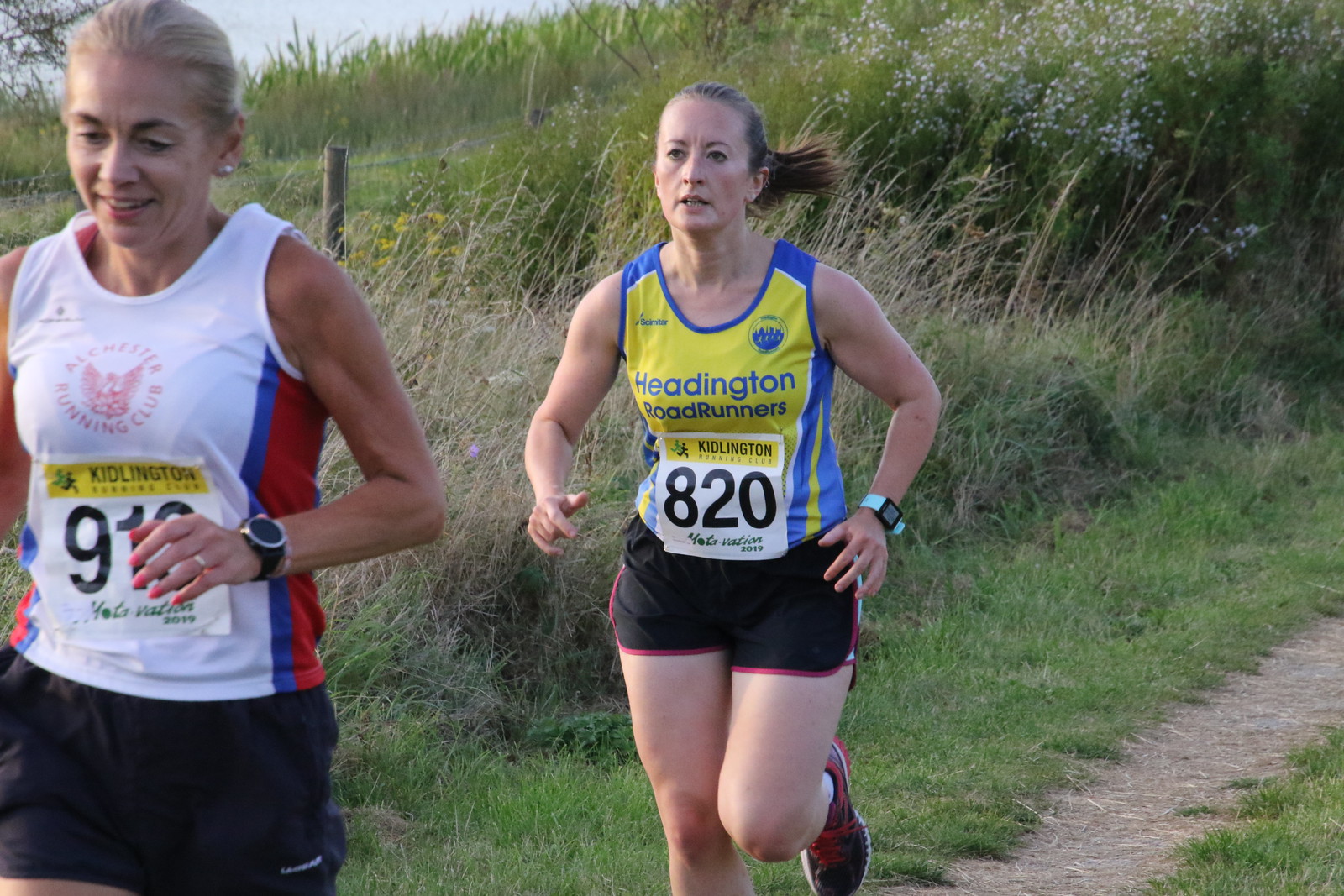The photograph captures two women running in what appears to be a race on a path surrounded by high grasses and wildflowers, including white, yellow, and possibly purple blooms. In the background, a solitary fence pole can be seen, hinting at more fencing along the route. The trail beneath their feet is a visible brown path interwoven with rich green shrubbery. 

The woman in the lead sports a black pair of shorts and a tank top labeled "Alchester Running Club." Her bib number starts with "91," though the last digit is obscured by her hand. She has blonde hair pulled back, pearl earrings, a watch, and a slight tan. The runner behind her, also in black shorts, wears a blue and yellow tank top reading "Headington Roadrunners" and has the bib number "820." She has brown hair pulled back, a watch, and a lighter tan, suggesting she might be a bit younger. Both women are running closely in line, showcasing their competitive stride amidst a scenic and natural backdrop.